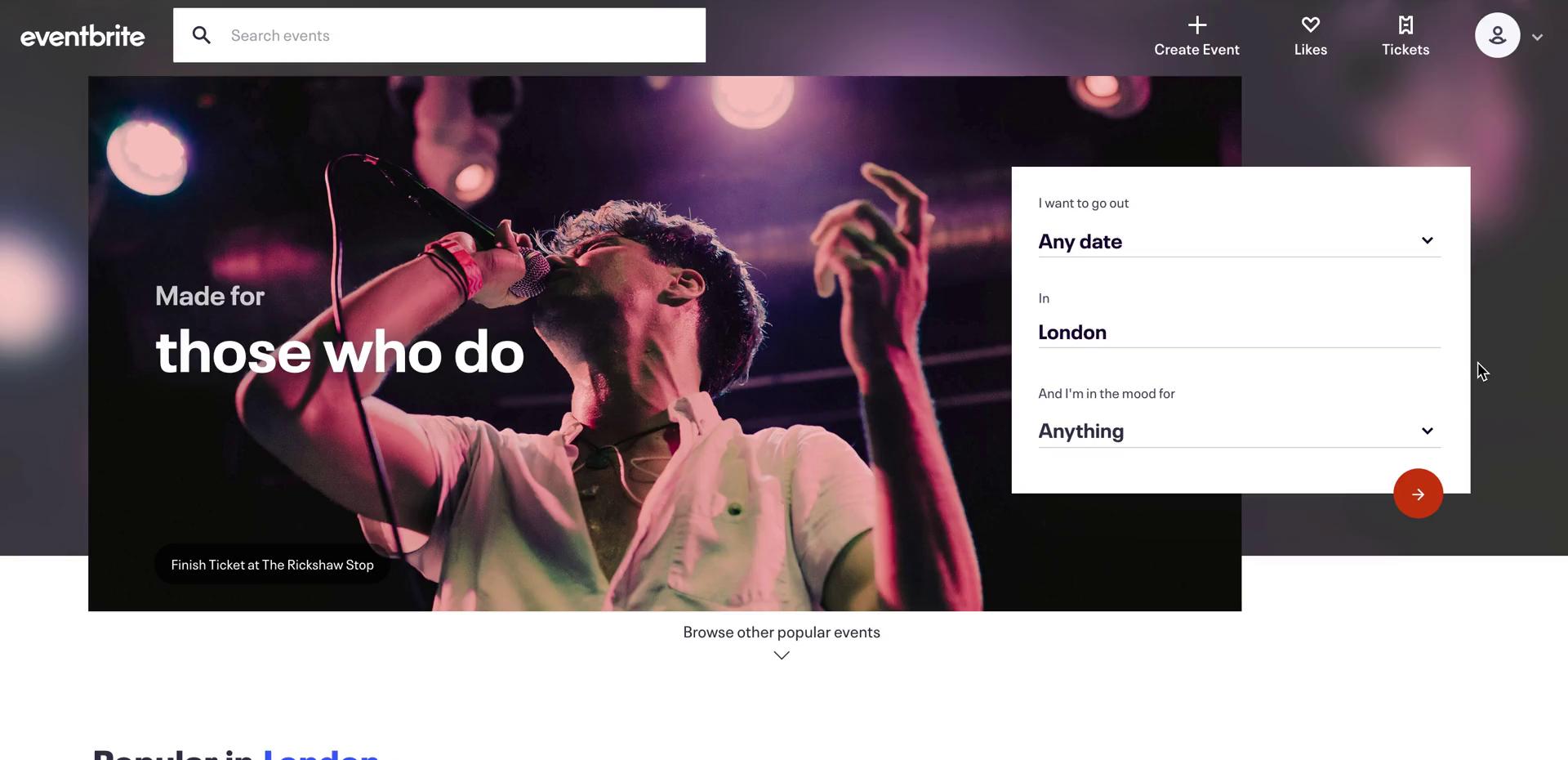This image is a screenshot from a webpage, with several distinct elements and an overall theme focused on event search and organization.

At the top left corner, the page features the logo "Eventbrite," and to its right are gray text prompts saying "Search events" within a white search bar that includes a dark gray magnifying glass icon. Adjacent to this, there are three clickable icons: a "Create" button marked with a plus sign, a "Likes" button denoted by a heart symbol, and a "Tickets" button represented by a ticket stub. Further to the right, there is a small white circle featuring an avatar icon with an arrow indicating further actions or menus.

Below this top navigation bar, there is a prominent image with motivational text stating, "This is made for those who do." The image depicts a performer passionately singing; he is raising one hand towards the sky while holding a microphone up to his mouth with the other hand. His face and eyes are partly obscured, though he is dressed in a white shirt and appears to be wearing a necklace and a wrist accessory, possibly a bracelet or watch on his right hand. The background showcases stage lights hanging from the ceiling. To the right of the performer, there is a text reading "Any date" and an additional, unspecified element labeled "One."